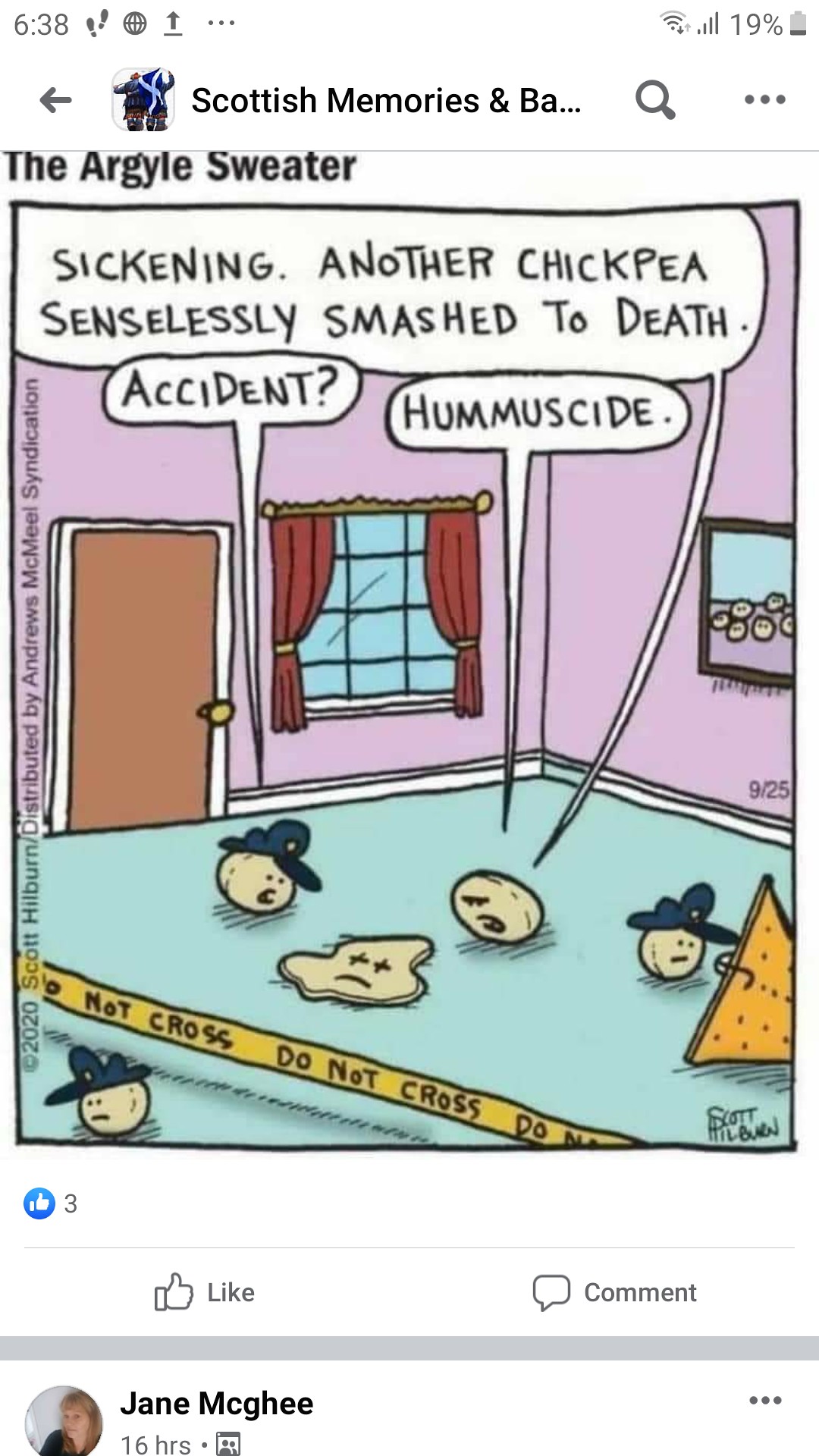The image is a screenshot taken from a mobile phone showing a Facebook post by Jane McGee. The time on the phone is 6:38, with the wireless signal at half strength, a fully loaded mobile signal pyramid, and the battery at 19%. The search bar at the top reads "Scottish memories." The post features a cartoon from "The Argyle Sweater" comic series, depicting a humorous crime scene inside a house with pink walls and blue floors. The scene includes several round-faced characters wearing hats amid a setting with yellow caution tape and a yellow triangle. Text bubbles above the characters read, "Sickening, another chickpea senselessly smashed to death," with one character saying, "Accident," and another replying, "Homicide," a play on the word "hummus." The post has three likes, indicated by a blue thumb icon, and includes like and comment buttons. Jane McGee's profile picture and name appear alongside the timestamp "16 HRS." The background beneath the post indicates it was shared on Facebook.